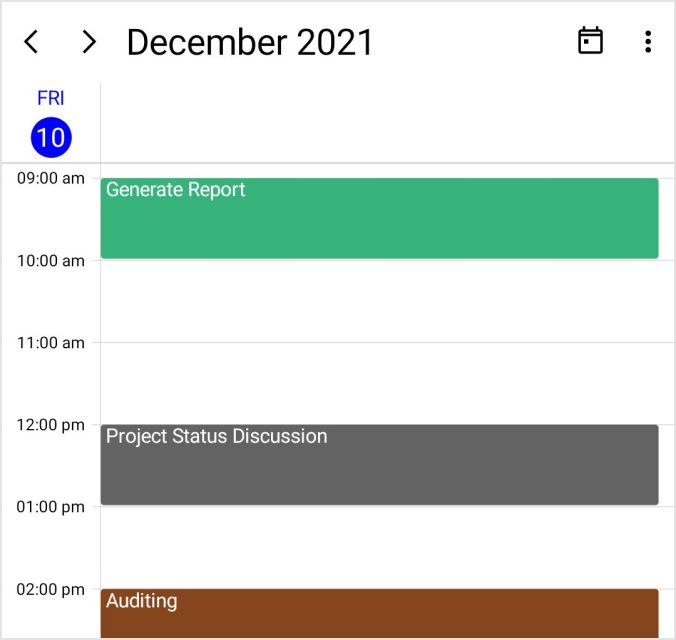The image captures a detailed daily schedule from a digital calendar, displayed on either a tablet or desktop screen without revealing the address bar, browser, or operating system details. 

In the top left corner, there are two black navigation arrows—one pointing left and the other right. The text "December 2021" is prominently displayed in black print. To its right, there is a small calendar icon followed by a vertical trio of dots indicating a menu for additional settings.

The date shown is Friday, December 10th, with "Friday" written in blue print. The "10" is displayed in white print within a small blue circle, signifying the current date.

The calendar shows a work schedule spanning from 9 a.m. to 2 p.m. The day begins with a green rectangular event labeled "Generate Report" from 9 a.m. to 10 a.m. Following this, there is a break until noon when a gray rectangle with white text marks "Project Status Discussion". Finally, at 2 p.m., a brown box signifies the "Auditing" task.

This thoroughly organized calendar provides a snapshot of a person’s workday on December 10th, 2021.